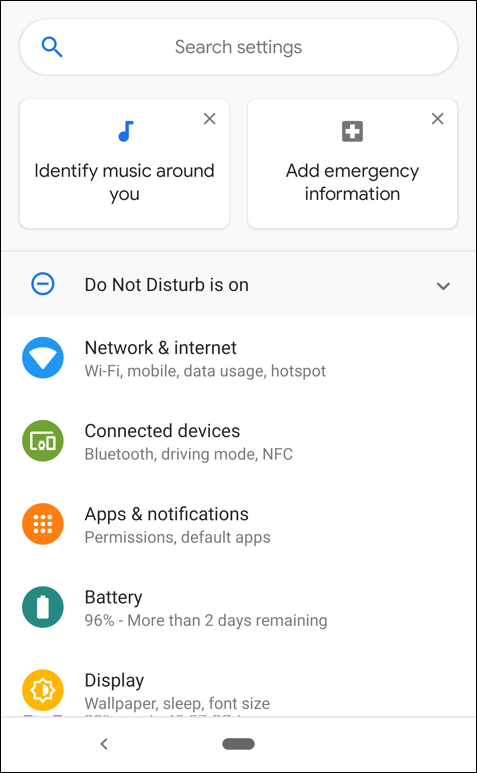The image showcases a smartphone settings interface against a light blue background. 

At the top, a white search box is presented with the phrase "Search settings" in light gray text. Below it, on the left, is another white box featuring a small blue music note icon and an "X" in the corner, accompanied by the text "Identify music around you." 

Beside this is a white box containing a black square with a white cross, labeled "Add emergency information," also with an "X" in the corner. Below these boxes, a horizontal line separates them from subsequent sections.

The interface continues with the "Do not disturb" option, marked as on, within a blue circle with a blue dash and a down arrow for more options.

Further down, the menu displays several sections on a white background:
- A blue circle with a white pie slice icon labeled "Network & internet," detailing Wi-Fi, mobile data usage, and hotspot options.
- A green circle with two white device icons, labeled "Connected devices," covering Bluetooth, driving mode, and NFC.
- A bright orange circle with nine white dots labeled "Apps," detailing app notifications, permissions, and default apps.
- A green circle with a white battery icon labeled "Battery," indicating 96% charge with more than two days remaining.
- A yellow circle with a white sun icon labeled "Display," covering wallpaper, sleep mode, and font size settings.

A gray dotted line and a gray left arrow are at the bottom, followed by a small black button surrounded by a light black line.

Overall, the detailed and color-coded sections efficiently organize various device settings for user navigation.